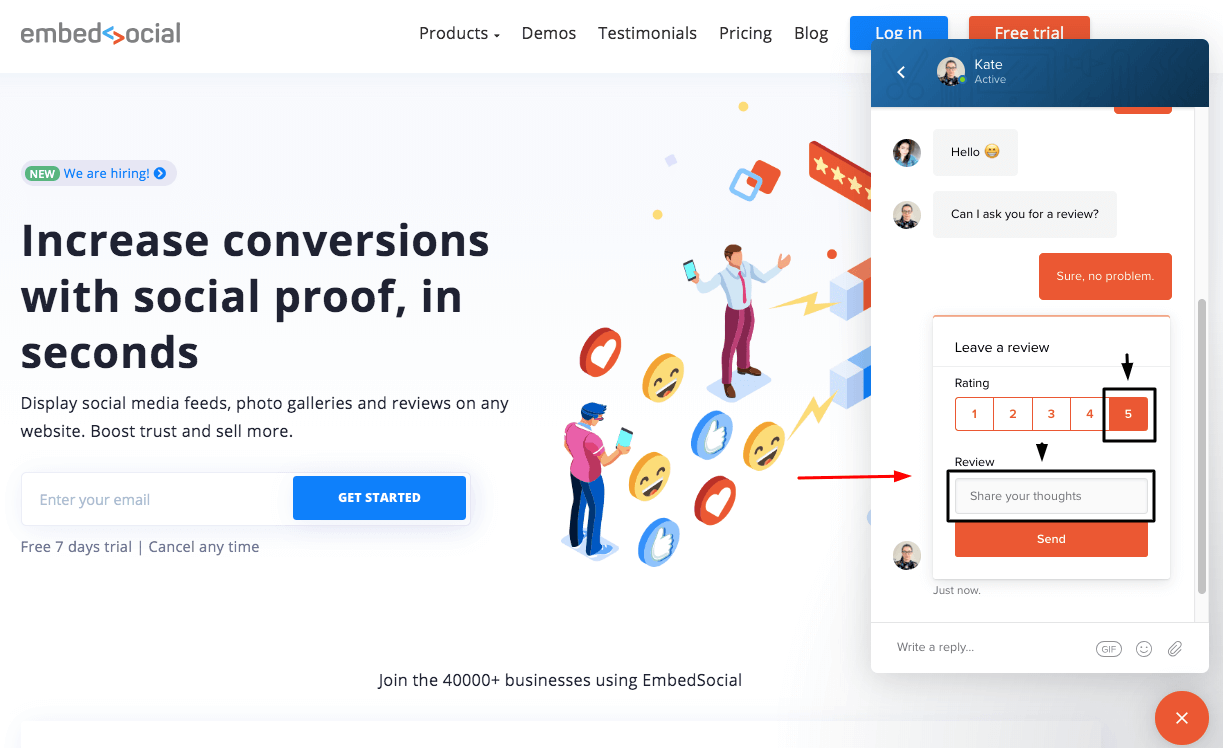### Detailed Descriptive Caption:

In the top left corner of a webpage, there is a logo for "Embed Social." The logo contains the text "Embed Social," where the 'S' is represented by two blue left arrows and two right orange arrows, creating a dynamic feel. 

To the right, the navigation bar includes links labeled "Products," "Demos," "Testimonials," "Pricing," and "Blog." A blue button labeled "Login" and an orange button labeled "Free Trial" are also present. 

Below the Embed Social logo, there is a small grey pop-up button featuring a green icon and text that says "New" and "We are hiring."

The main banner beneath this section reads, "Increase Conversations with Social Proof." This headline is supported by additional text suggesting users can "Display social media feeds, photo galleries, and reviews on any website to boost trust and sell more." 

A call-to-action box below this encourages users to "Send your email," featuring a blue button with white text that says "Get Started." A note below the button informs users of a "Free seven-day trial" with the ability to cancel anytime.

To the right, there is an engaging image featuring two men surrounded by several emojis and a star rating. Further to the right, a blue box at the top reads "Kate Active," alongside a picture showing a conversation where one person asks, "Hello, can I ask you for a review?" Prompting the user with an orange button that says "Sure, No Problem. Leave a Review." A star rating selector and a text box invite users to "Share your thoughts," ending with an orange button labeled "Send."

In the bottom right-hand corner, a distinct orange circle with a white 'X' serves as a close button for the pop-up or embedded feature.